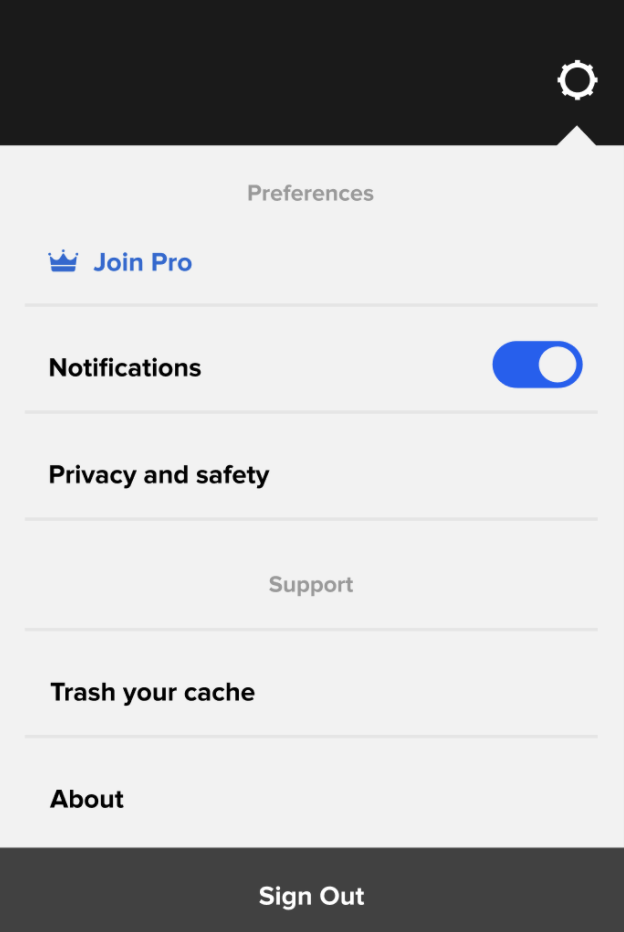The image portrays a detailed view of an application's preferences screen. At the top right corner, there's a cogwheel icon symbolizing the settings menu, highlighted by a small triangle pointing towards it. Directly below the preferences heading on the left side, there's an illustration of a blue crown beside text that reads "Go Pro," also in blue. Following this section are several headings in black text, starting with "Notifications," which is accompanied by an enabled slider on its right. Next, the "Privacy and Safety" section is displayed. Moving downwards, the support section is marked by a central gray heading labeled "Support." Under this heading, the options "Trash Your Cash" and "About" are listed in black text on the left side. At the very bottom of the image, the word "Sign Out" is presented in white text on a gray panel.